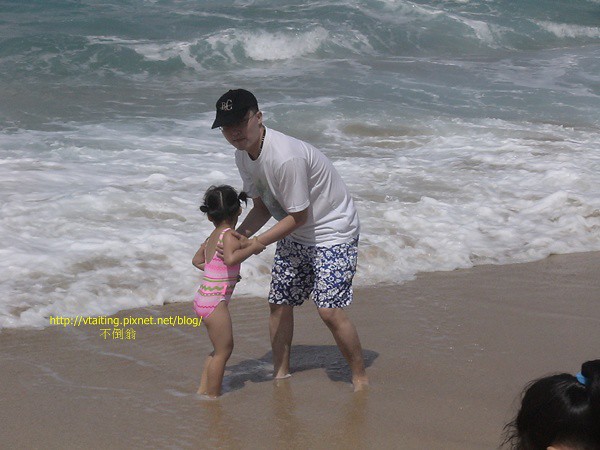In this compelling beach scene, a man in a white t-shirt adorned with flower-patterned beach shorts and a black cap attempts to lift a baby girl wearing a pink swimsuit just by the shore. The baby girl, with dark, pigtailed hair, gazes out towards the waves, creating a picturesque moment against the backdrop of frothy white surf and darker gray seawater. The man's head is turned towards the camera, revealing his glasses, while a barely noticeable yellow text, "http://biting.picsnet.net/.blog/," overlays the image. Adding depth to the composition, a small wave is visible around 20 feet from the shore, enhancing the coastal ambiance. In the lower right corner, the head of another girl with dark hair and a blue ponytail holder subtly intrudes, amplifying the sense of a lively day at the beach.